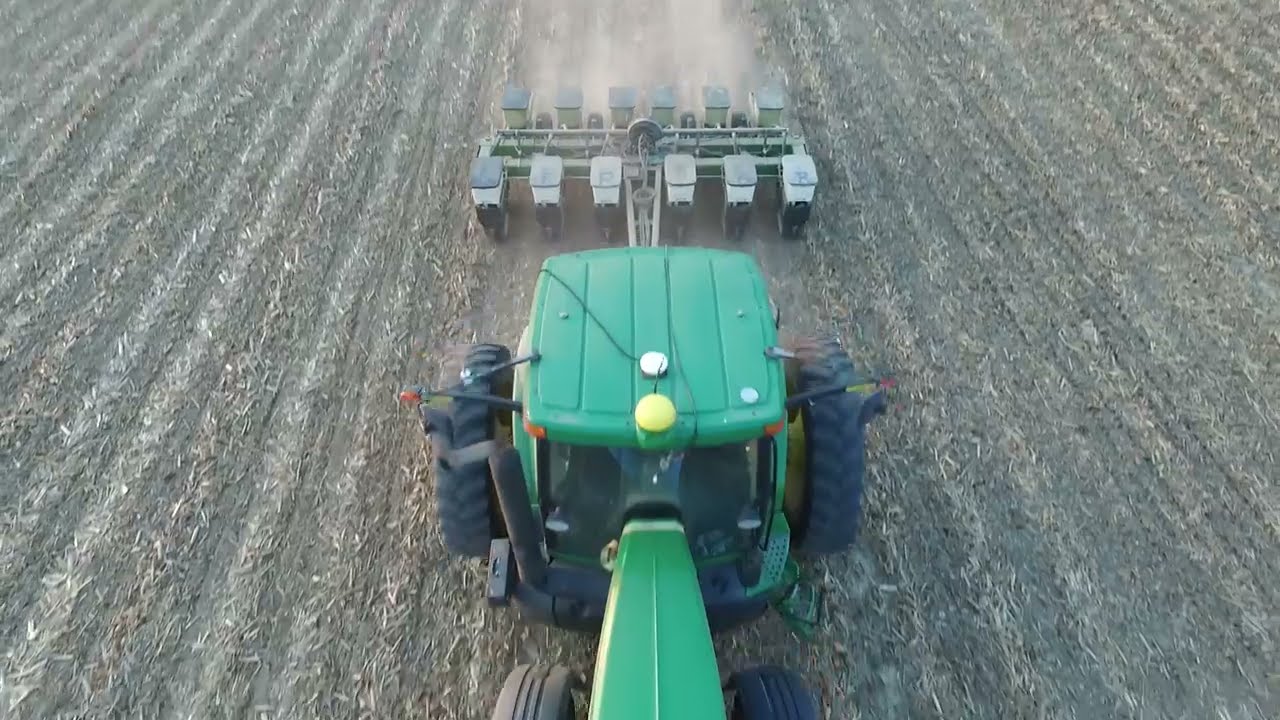This aerial, photorealistic image captures a farming scene during what appears to be late afternoon or early evening, as indicated by the soft lighting. The focal point is a green tractor, roughly centered and heading toward the viewer, with the front partially obscured. It features black wheels, smaller at the front and larger at the back, with distinctive yellow hubs. The tractor is traversing a dry, brownish field filled with straw, hay, and crushed crop residue. Attached to the tractor is a sizable green machine with two sets of six white hubs on either side, trailing a cloud of brown dust. A small patch of green grass peeks through in the top left corner, providing a slight contrast to the otherwise earth-toned landscape. The image doesn't feature any text, and the tractor's cabin interior is only partially visible, with no clear view of the driver.